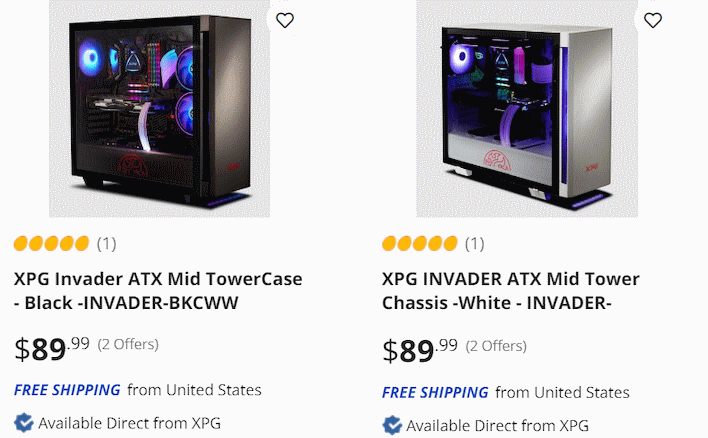This image showcases a sales page featuring two computer tower cases, presented in two square boxes. The first box displays the "SPG Invader ATX Mid-Tower Case" with sleek black brushed sides. It features a red logo at the bottom of the case, and has received one review, boasting a five-star rating. The product is priced at $89.99, with free shipping from the United States, and is available directly from XPG.

The second box features a similar "XPG Invader ATX Mid-Tower Chassis" but with sophisticated aluminum brushed sides. This case also sports a bright red logo at the bottom. Like the first, this case is priced at $89.99. It mentions there are two offers available, and also includes free shipping from the United States, available directly from XPG.